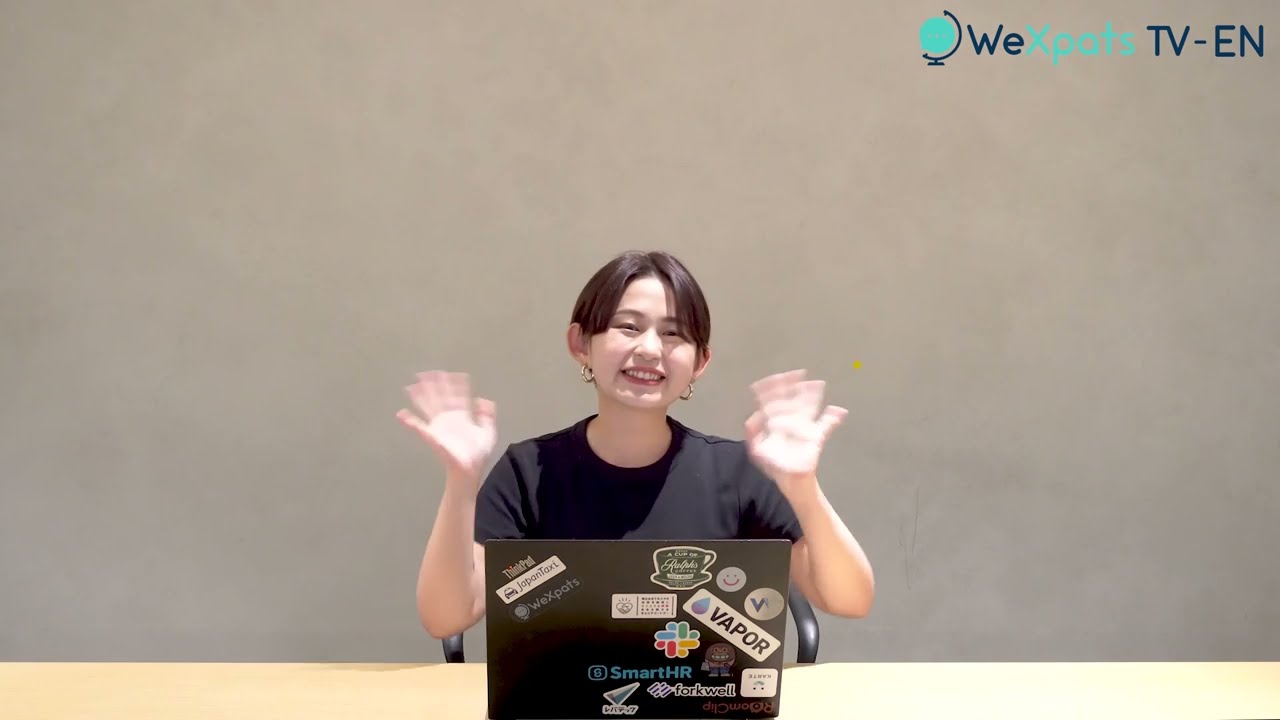This is a detailed photograph of a smiling woman seated at a light brown wooden desk, indoors. She has short brown hair and is wearing small gold hoop earrings and a plain black short-sleeved t-shirt. In front of her on the desk is a black laptop adorned with various stickers including ones that say "WeExpats," "Vapor," "SmartHR," an image of a coffee cup, and a smiley face. The woman is waving her hands, which appear slightly blurry due to their motion. The background features a gray wall, and in the upper right corner, there is text that reads "WeExpats TV-EN" with a logo of a spinning globe next to the text.